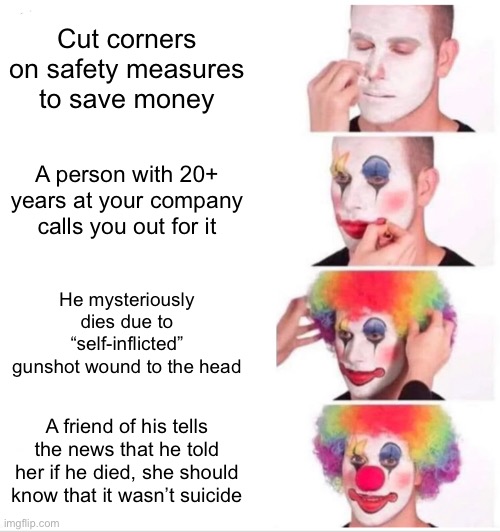The image is divided into eight sections: four on the left side and four on the right side. On the left side, each section features a white background with black text. On the right side, a person is shown transforming into a clown.

Top left section: The text reads "Cut corners," followed by "on safety measures," then "to save money."

On the right side, the first image shows a close-up of a person's face in a black t-shirt, applying white makeup as a base.

Middle left section: The text continues with "A person with 20+ years," followed by "at your company," then "calls you out for it."

The second image on the right shows the person with red lips and colored eyebrows - one blue, one yellow.

Bottom left section: The text reads "He mysteriously dies," followed by "from a self-inflicted gunshot to the head."

The third image on the right shows the person with a rainbow-colored wig, featuring red, orange, yellow, green, blue, and violet.

Final left section: The text reads "A friend tells the news," followed by "he told her if he died," then "she should know it was a suicide."

The final image on the right shows the clown transformation complete: the person has a red nose, red mouth outlined in black, and is looking directly at the camera.